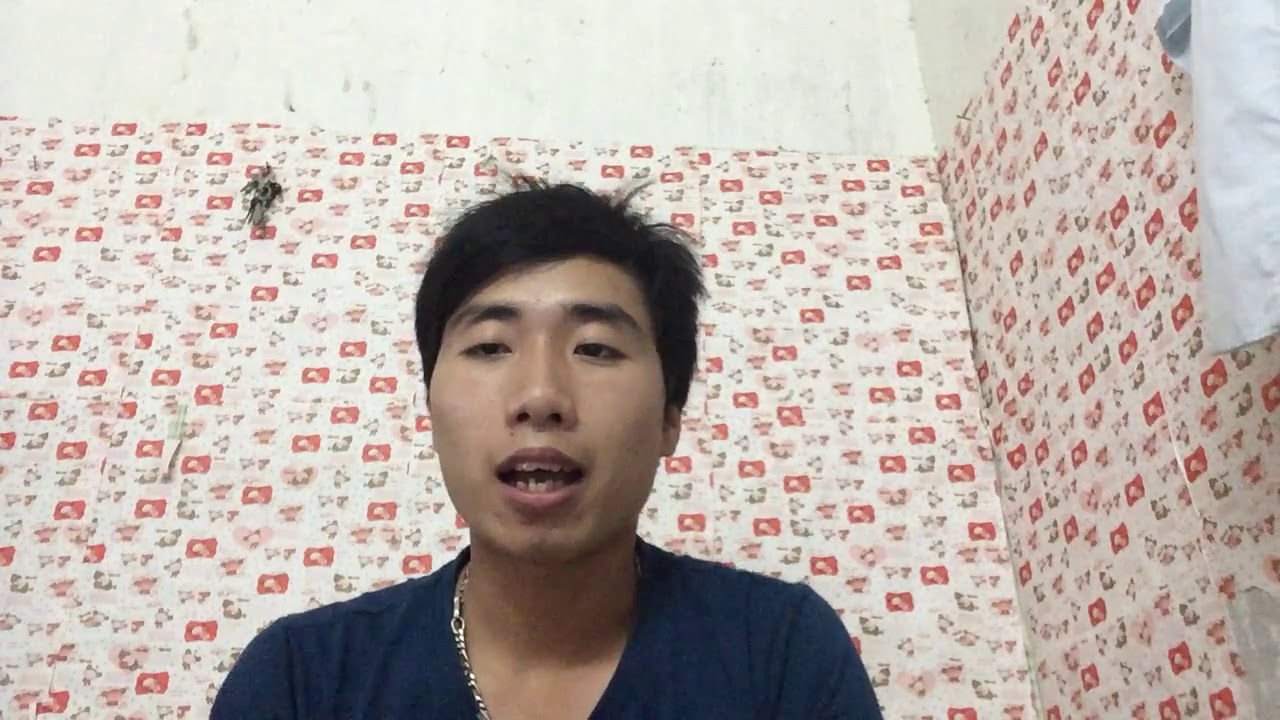This photograph, styled in a realistic, indoor setting, features a young Asian man in his 20s or 30s, with black hair and a slightly open mouth as if talking to someone. He wears a black shirt and a silver necklace, with notably jagged teeth. The man is positioned in a corner of a room, in front of a distinctive wall. The lower part of the wall is adorned with wallpaper that extends two-thirds up and features red logos or designs on an off-white background, while the upper part is white, albeit somewhat dirty. The wallpaper appears slightly old or possibly peeling in places. To the right of the subject, a towel hangs from a rack, adding a homely touch. Despite some differing opinions on minor details, the homey environment and the expressive posture of the man stand out clearly in the image.